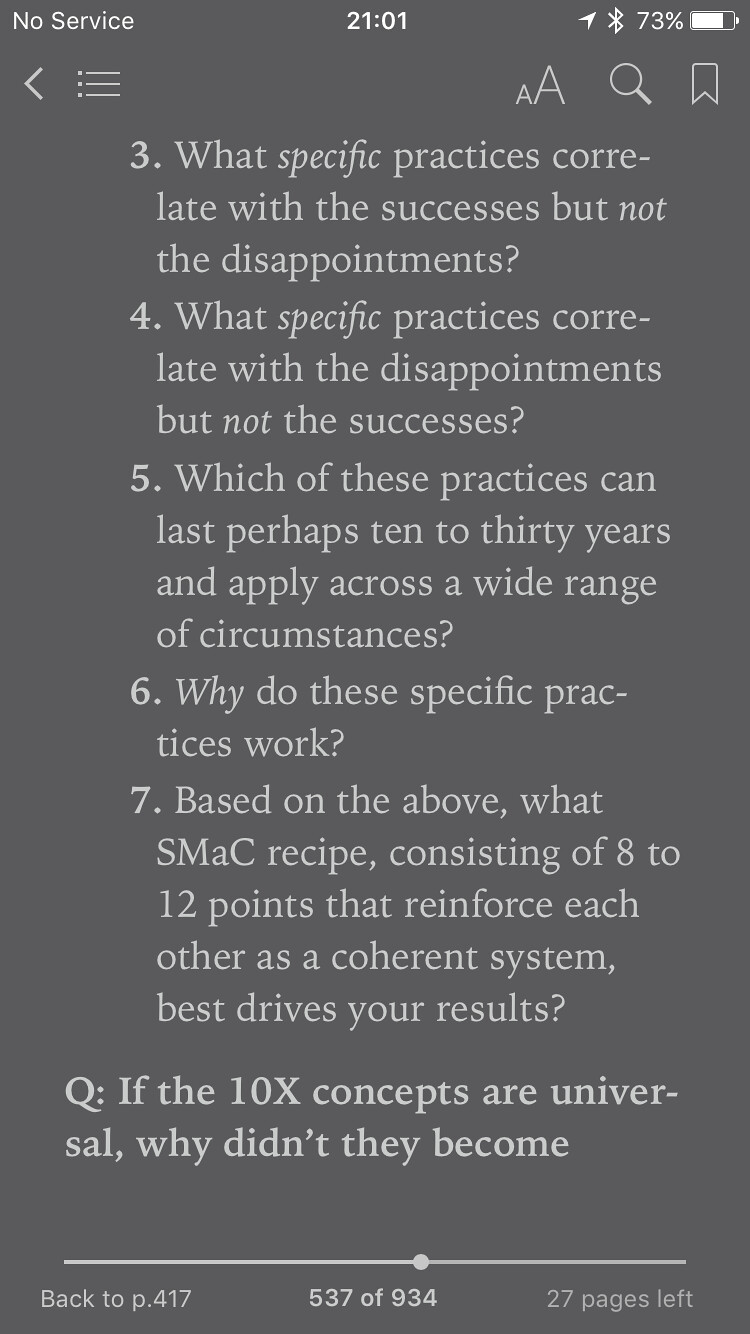This image is a detailed screenshot taken from the Books app on an iOS device. The screen displays a gray background with white text, presenting a series of questions that seem to delve into specific practices associated with successes and disappointments. At the top left corner, the status bar indicates "No Service," while the center shows the time as 21:01, and the top right shows a Bluetooth icon and a battery status of 73%. Below the status bar, there are icons for navigation, including a left arrow, menu options, text size adjustment, a magnifying glass for search, and a bookmark icon.

The main text on the page reads:
1. What specific practices correlate with the successes but not the disappointments?
2. What specific practices correlate with the disappointments but not the successes?
3. Which of these practices can last perhaps 10 to 30 years and apply across a wide range of circumstances?
4. Why do these specific practices work?
5. Based on the above, what SMAC recipe consisting of 8 to 12 points that reinforce each other as a coherent system best drives your results?
6. Question: If the 10x concepts are universal, why didn’t they become...

At the bottom of the screen, a navigation bar indicates the user's current position in the book: "Back to page 417" on the left, "537 of 934" in the center, and "27 pages left" on the right. The scrubber bar helps indicate the reader's progress. The comprehensive nature of the questions implies a focus on long-lasting, widely applicable successful practices.